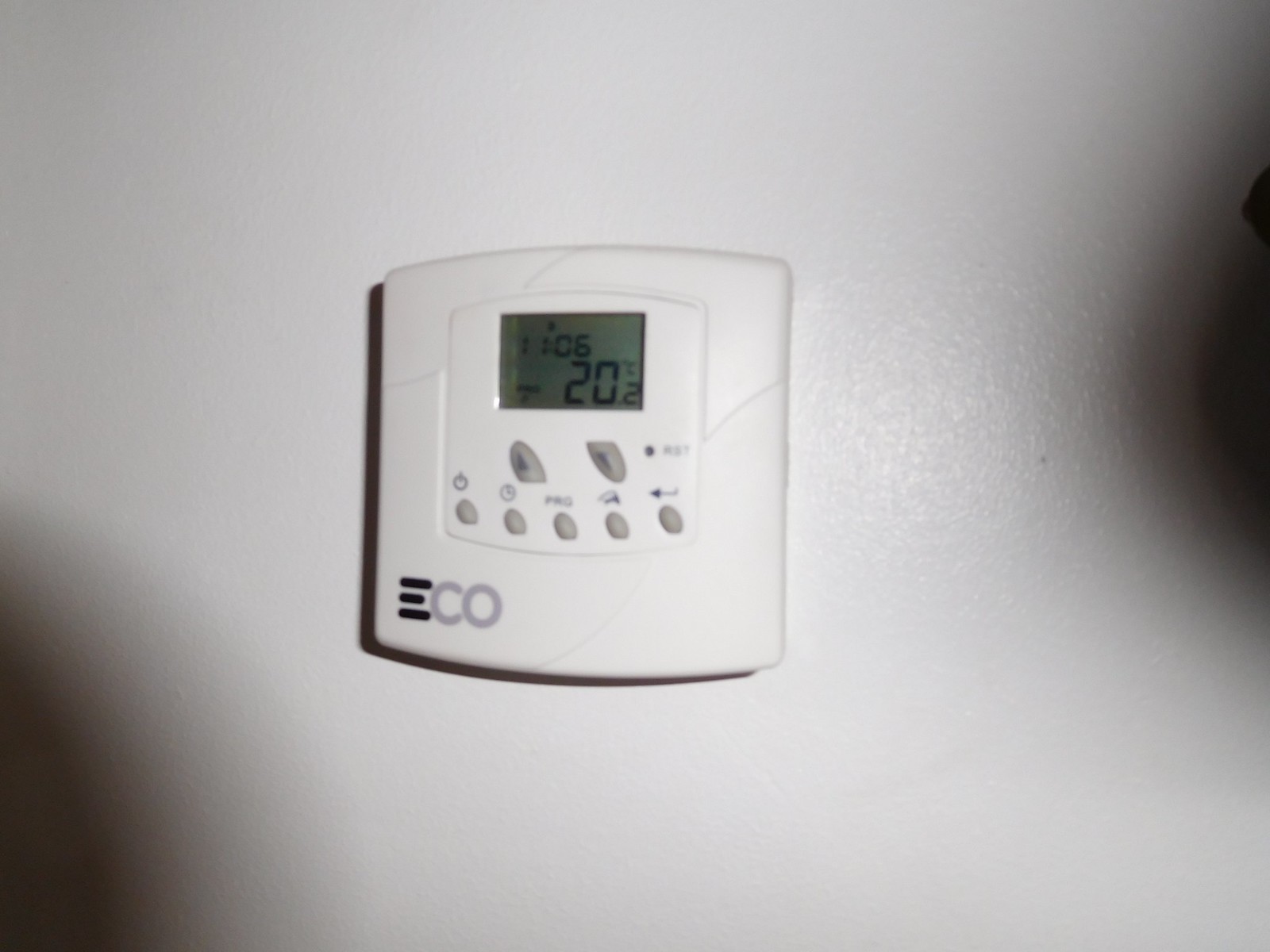The photograph captures a detailed view of a wall-mounted thermostat positioned against an older-type, white-painted drywall. The wall lacks any stucco texture, and the paint reflects light in a particular way that suggests an older drywall material. The lighting creates two distinct circular shadows, one on the bottom left and another on the right side of the image, possibly from hands or objects held out of frame.

The thermostat itself is a medium-sized, white square device. Notably, "CO" is marked in gray on the bottom left of the device, which is likely the brand name. The thermostat's design features include three black lines on the bottom left and additional horizontal lines across the left, right, and top edges.

Prominently integrated into the thermostat is a smaller, nearly square component with rounded edges. At the top of this section is an old-fashioned screen with a grayish-green hue, typical of older electronic displays. The screen displays the time "11:06" and the temperature reading "20°C." Below the screen are two larger gray buttons on either side designed for adjusting the temperature. Further down, there are five smaller gray buttons for power, settings, and other functionalities, among which is a reset button positioned directly under the screen.

Overall, the thermostat showcases multiple options and settings, offering both traditional and advanced user interactions in a somewhat dated but functional design.